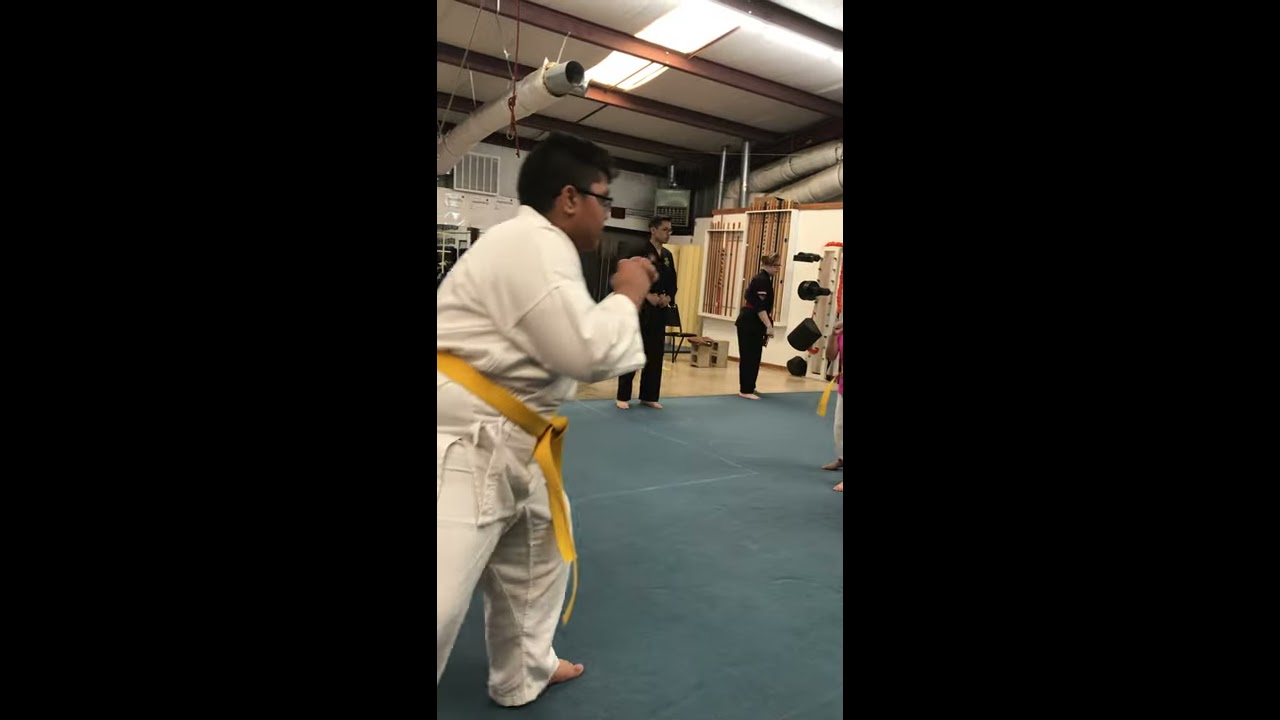In the image, an overweight boy with short black hair, glasses, and tan skin is seen in the foreground, standing on a large, dull blue mat. He is wearing a white karate gi adorned with a yellow belt tied around his waist. His arms are raised in a fighting stance, with his left leg lunging forward. The setting appears to be a martial arts studio, characterized by its industrial ceiling that has brown metal beams, HVAC vents, and lights. In the background, two adults dressed in black karate uniforms observe the scene. One of the instructors is male and the other female, and both seem focused on the boy's practice. Various martial arts memorabilia are visible in the studio. The image is framed by large black borders on the left and right sides.